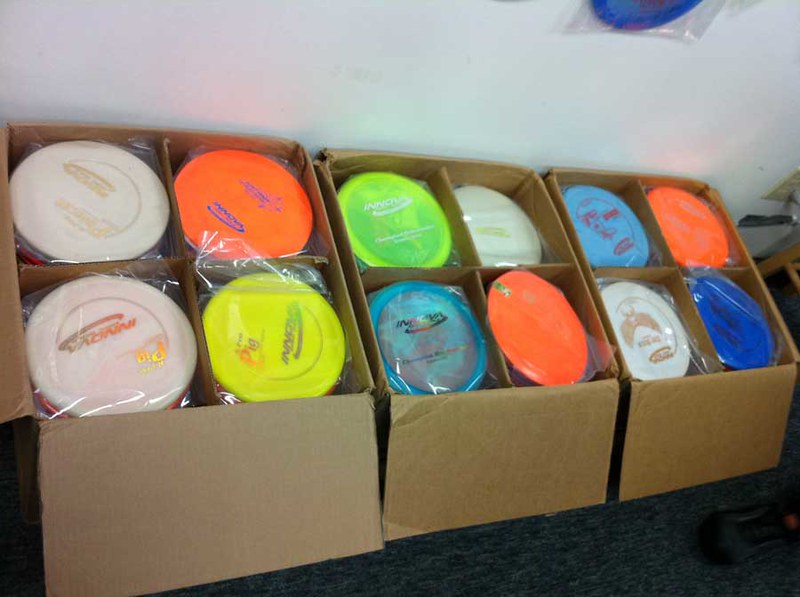The photo depicts a top-down view of three open cardboard boxes, each divided into four compartments, sitting on a dark gray surface with a white wall in the background. Each compartment contains a different colored frisbee, meticulously arranged in a repeating pattern. From left to right, the frisbees display a rotation of colors including cream, orange, yellow, neon green, and various shades of blue. Specifically, in the leftmost box, the sequence starts with two cream-colored frisbees, followed by an orange, yellow, neon green, and blue frisbee. In the middle box, the colors are neon green, blue, cream, and orange. The box on the far right showcases light blue, dark blue, cream, and orange frisbees. Notably, the frisbees feature distinctive writing in colors matching their backgrounds; white frisbees have gold writing possibly spelling "I-N-N” or “O-D-V-A,” orange ones have blue writing, and the neon green frisbees display either gold or silverish writing, while some green frisbees have white writing. The organized arrangement suggests these frisbees are ready to be stocked onto a store floor. Additionally, a small portion of a brown stool is visible at the right center of the image.